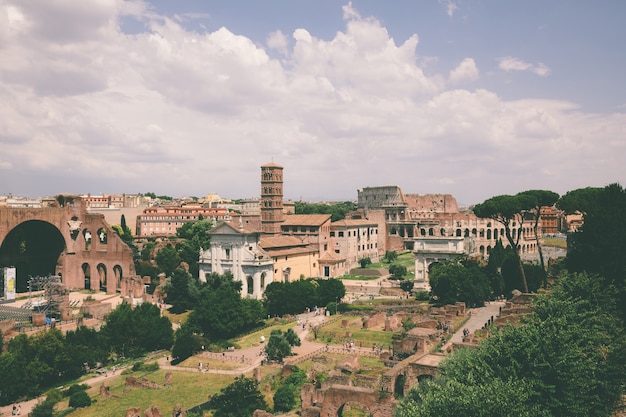This exterior photo captures an ancient European cityscape, potentially Rome, showcasing a blend of ruins and historic buildings crafted from neutral brown and white stone and brick. The foreground reveals the remains of a building, which opens up to a grassy courtyard encircled by dark green trees, shrubs, and bushes. A road or walkway runs along the bottom center right, beside a cluster of tree tops. The perspective is from a slight overhead vantage point, giving prominence to the grassy area in the foreground and the buildings receding into the background.

Prominently, an arched entrance on the left-center side stands in shadow, leading the eye to the city's towering structures. In particular, a block-style tower, several stories high, dominates the central background. To the right side, the distant silhouette of the Colosseum suggests the location might be Rome, reinforcing the sense of ancient grandeur. The landscape features gently rolling hills beyond the city, enhancing the historical atmosphere.

In the sky, a mix of white and gray-toned clouds stretch from left to right, with patches of blue peeking through in the upper right corner to the center. The image captures a dynamic and historically rich milieu, with modern visitors walking along designated paths, indicating its status as a contemporary tourist attraction.